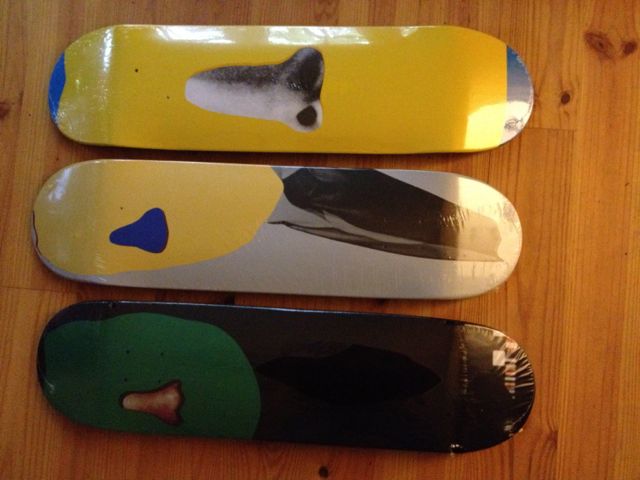This color photograph depicts three snowboards placed horizontally in a row on a medium wood-colored floor, showcasing its grain, lines, and distinct character. The wooden surface is illuminated from the right side, suggesting a nearby light source.

The top snowboard is predominantly yellow with blue accents at the ends. It features a black-and-white photograph of a person's nose in the middle. The second snowboard is primarily yellow and gray, with a small blue nose-shaped object within the yellow section and an additional black element. The third snowboard is mostly black with a green section on the left end, which includes a color photograph of a person's nose. The detailed visual elements of the snowboards and the rich texture of the wooden floor provide an intriguing and textured composition.